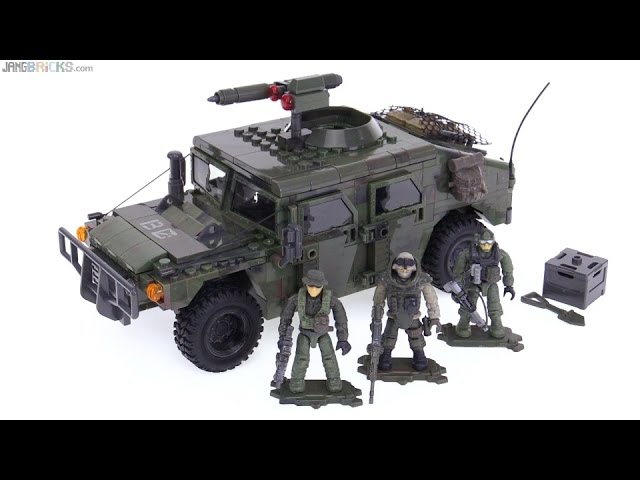The image features an intricate Lego military set, showcasing a detailed military hummer as its centerpiece. The hummer is robustly designed, equipped with armor plating and an array of weaponry, including a missile launcher mounted on top. Positioned in front of the hummer are three action figures, each geared up in body armor and brandishing weapons, clearly prepared for combat scenarios. These figures are designed to fit inside the hummer, allowing for versatile play where they can be transported and then deployed for battle missions. Additionally, the set includes a supply box filled with various essential items, likely intended to support the action figures in their operations. Overall, this dynamic and engaging toy set promises hours of imaginative play for children interested in military-themed adventures.